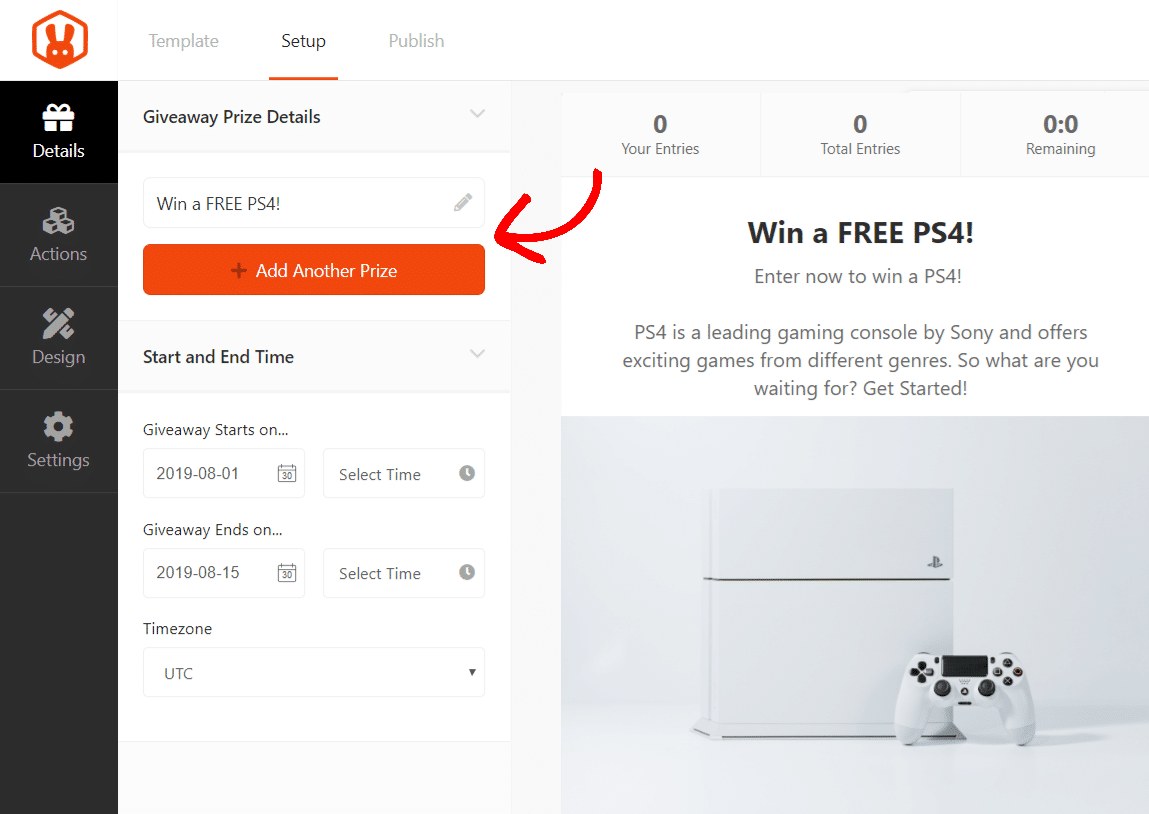**Caption:**

The screenshot displays a webpage layout for organizing a giveaway contest. In the upper left-hand corner, there is a hexagon icon featuring an orange bunny with upright ears. The current section, indicated by a black template button with an orange outline, is selected. Nearby, a primary "Publish" button allows the user to finalize their contest setup.

On the left-side menu, a variety of options are available, each with distinct black icons and white text descriptions:
- "Details" – represented by a gift icon.
- "Action" – depicted with three cubes.
- "Design" – shown with a crossed pencil and ruler.
- "Settings" – illustrated with a cogwheel.

At the top of the main content area, a section titled "Giveaway Prize Details" includes a dropdown menu for selecting the prize, which in this case is a "Win a free PS4." An orange button labeled "Add Another Prize" in white text is prominently displayed, highlighted by a red arrow.

Further down, fields are provided to specify the start and end times of the giveaway:
- Start date: 2019-08-01.
- End date: 2019-08-15.
- Time zone: UTC.

On the right-hand side of the page, there's a status panel showing:
- Your entries: 0.
- Total entries: 0.
- Remaining: 0 of the available entries.

In bold text, the prize is advertised as "Win a free PS4," encouraging users to "Enter now to win a PS4." The PlayStation 4, described as a leading gaming console by Sony offering exciting games across various genres, is visually represented with an image of a white PS4 and a matching controller against a white background.

Overall, the page appears to serve as a comprehensive interface for setting up and managing a giveaway contest.